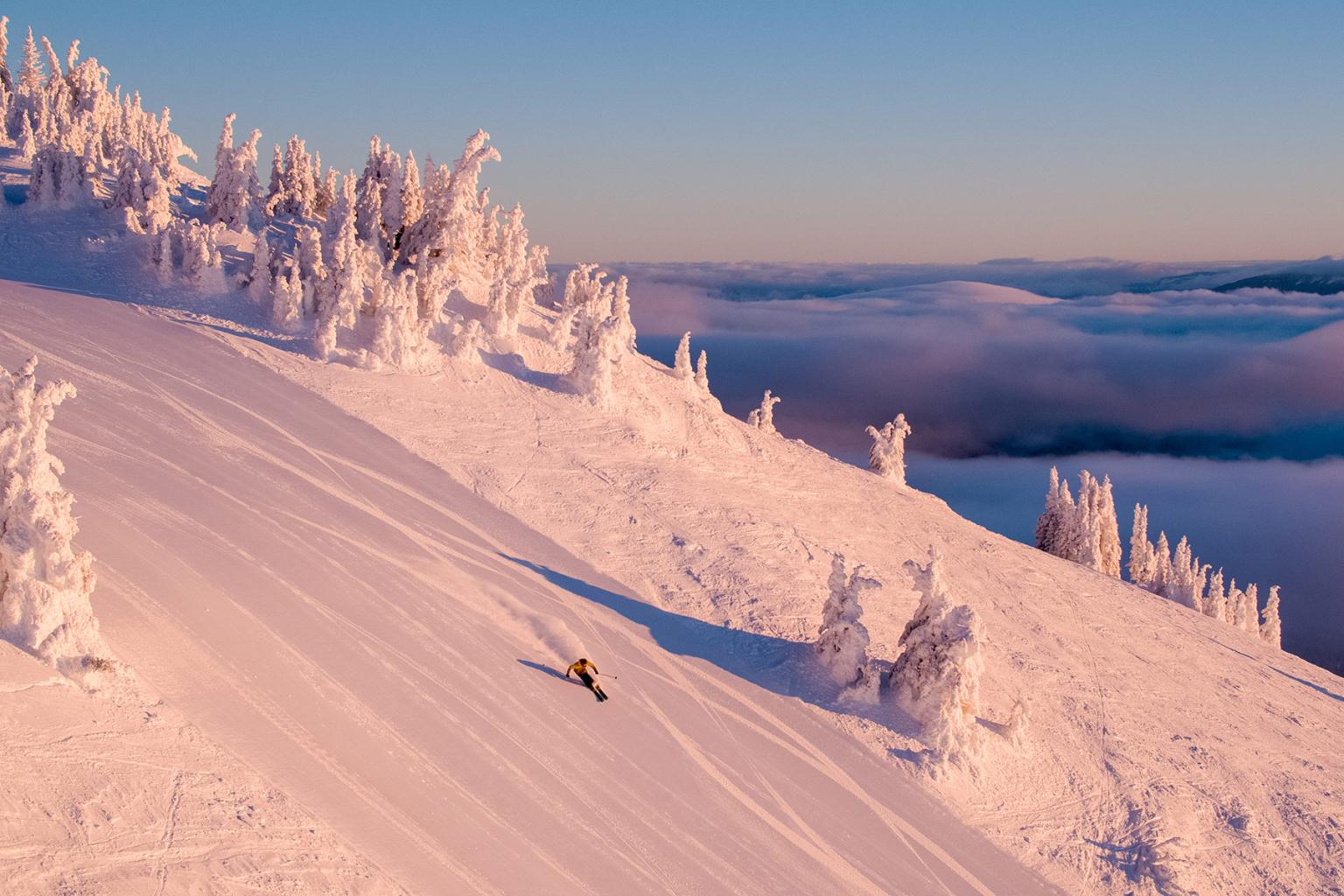The image is an aerial photograph of a snow-covered ski slope taken from a high vantage point, possibly from a drone or a high overlook on a mountain. The central focus of the image is a skier dressed in an orange top and black pants, navigating down the smooth, white expanse with black skis. A small snow drift follows the skier, highlighting their motion. The slope, marked by various ruts and lines from previous descents, runs diagonally from the center left to the center bottom of the photograph. Flanking this main track are slightly upward sloping areas dotted with small pine trees heavily laden with ice and snow. In the upper right portion of the image, the mountain reaches such a height that it towers above the cloud cover, revealing a clear blue sky that transitions into a muted orange hue near the horizon, indicating a possible sunrise or sunset.